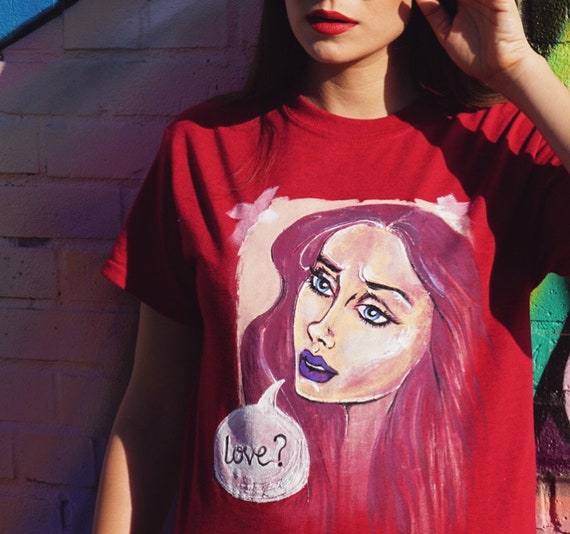This photograph features a young Caucasian woman standing against a rugged and colorful brick wall that blends shades of purple, lilac, blue, white, tan, green, lime, and coral. The image is cropped to show her from just below her nose to her waist, so her eyes and nose are not visible. She sports bright red lipstick and is dressed in a short-sleeved red t-shirt that prominently displays a drawing of another woman. This illustrated woman has long reddish-purple hair, green eyes, and blue lipstick. She appears to have a concerned expression and a white speech bubble emerging from her mouth that reads "Love?" in black script.